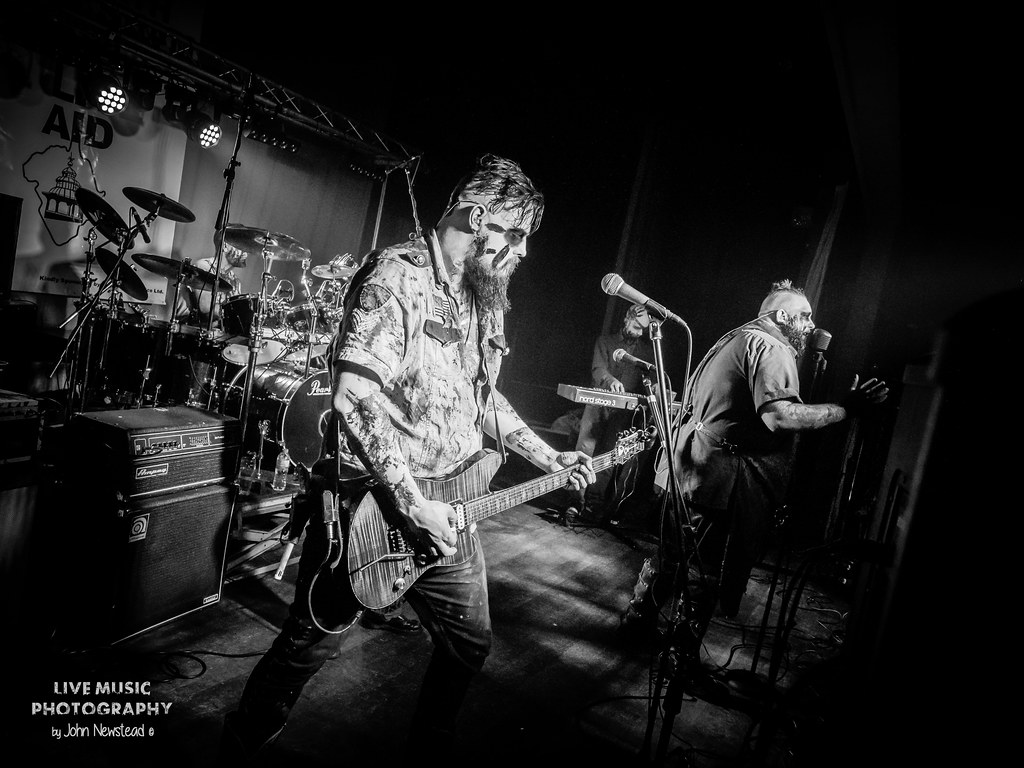This striking black, white, and gray photograph, professionally captured and credited to "Live Music Photography by John Newsted" in the bottom left corner, showcases a band mid-performance on stage. Dominating the center foreground is a guitarist with slicked-back, partially face-painted hair and a shaggy beard, clad in a short-sleeved, military-style shirt and jeans. His guitar features a notable striped woodgrain pattern. Next to him, a larger man, sporting a mohawk and equally shaggy beard, fervently sings into a vintage condenser microphone. The background reveals several more details: a sign reading "Aid" possibly indicating a charitable cause, a bald keyboardist with a handprint design on his head plays discreetly at the far back, nestled among speakers and subwoofers. Though barely visible, a drummer can be faintly made out behind an elaborate drum kit. The photograph expertly encapsulates the intensity and intricacies of a live musical performance.